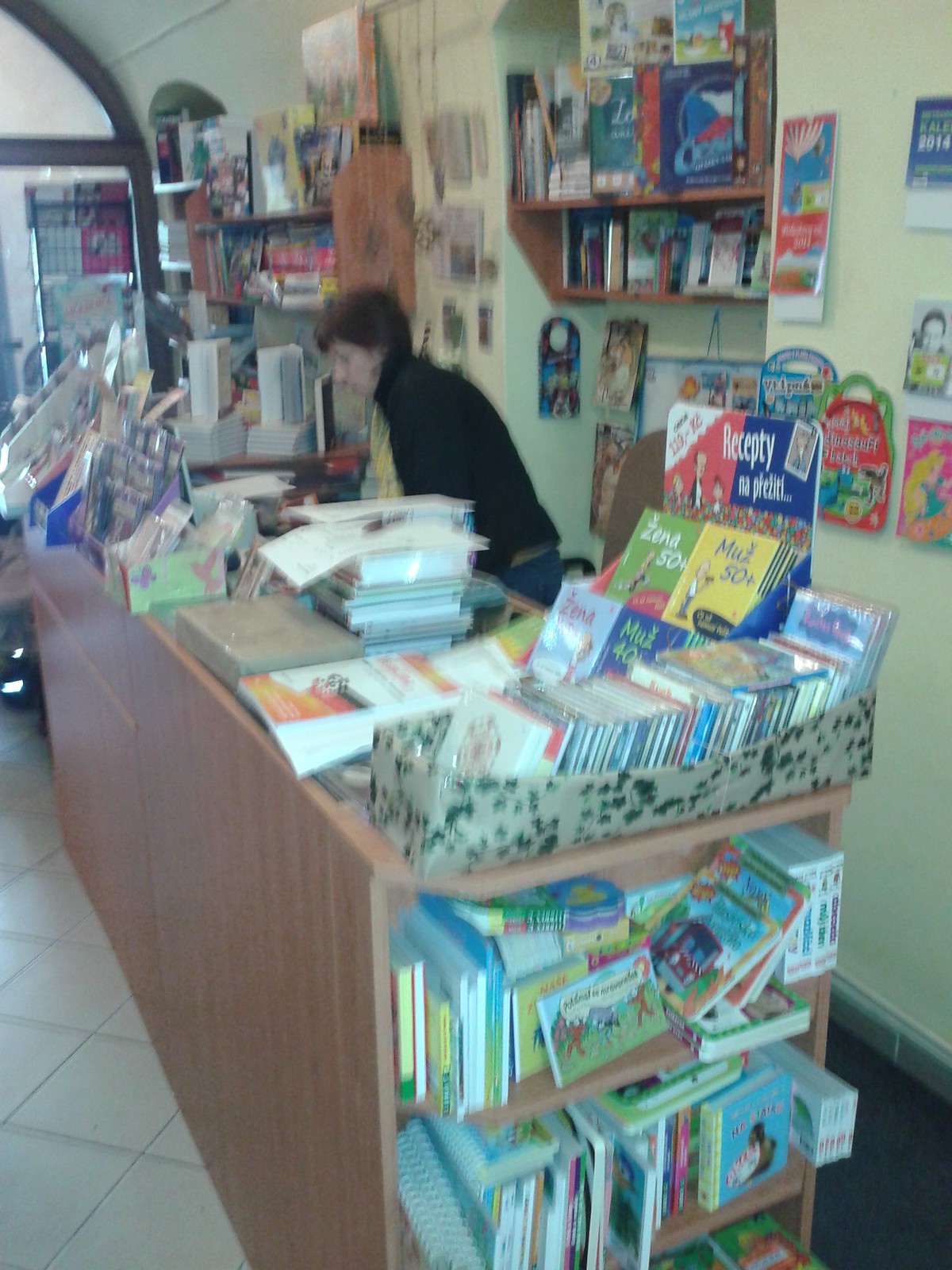The image depicts a cozy bookshop filled with an array of colorful books. Though the image is blurry, one can clearly discern the shopkeeper, dressed in a red top and blue pants, standing near a counter overflowing with books. Shelves crammed with books line the lower part of the image, and additional shelves filled with books are visible on the wall behind the shopkeeper. A brown box rests on the cluttered countertop. In the top left corner, a black archway door stands out against the white walls, while the cream-colored floor adds a warm tone to the shop's atmosphere.